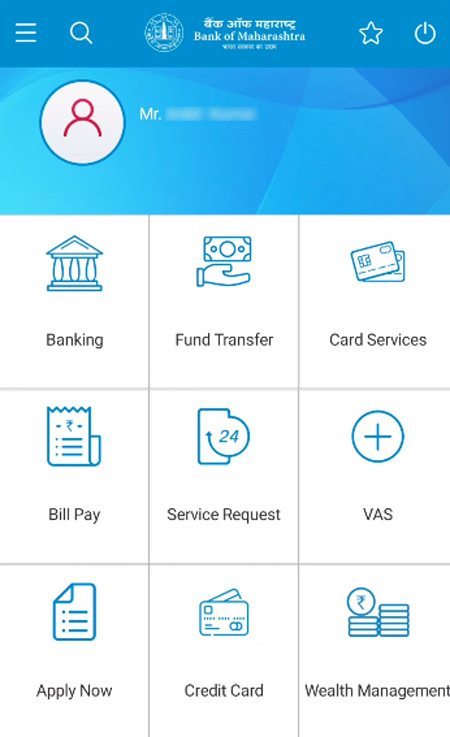The screenshot displays the homepage of the Bank of Maharashtra website. At the top, it prominently features the bank's name and logo. There's a user profile section labeled "Mr. Somebody," though the personal details are blurred out for privacy. The interface includes various navigation buttons such as a menu button, search button, favorites button, and a power button for logging in and out.

Beneath the header, the site offers a variety of categories for user navigation:
- **Banking:** Represented by an icon of a bank building.
- **Fund Transfer:** Illustrated with an image of a hand holding a bill.
- **Card Services:** Denoted by an icon of credit cards.
- **Bill Pay:** Shown with a receipt icon.
- **Service Request:** Indicated by a 24-hour availability icon.
- **Apply Now:** Presumably for new applications.
- **Credit Card:** Likely specific to applying for a credit card.
- **Wealth Management:** Marked by icons of stacked coins.
- **VAS (Value Added Services):** Represented by a circle with a plus sign.

The webpage is designed to facilitate easy access to various banking services via clearly labeled and intuitive icons.